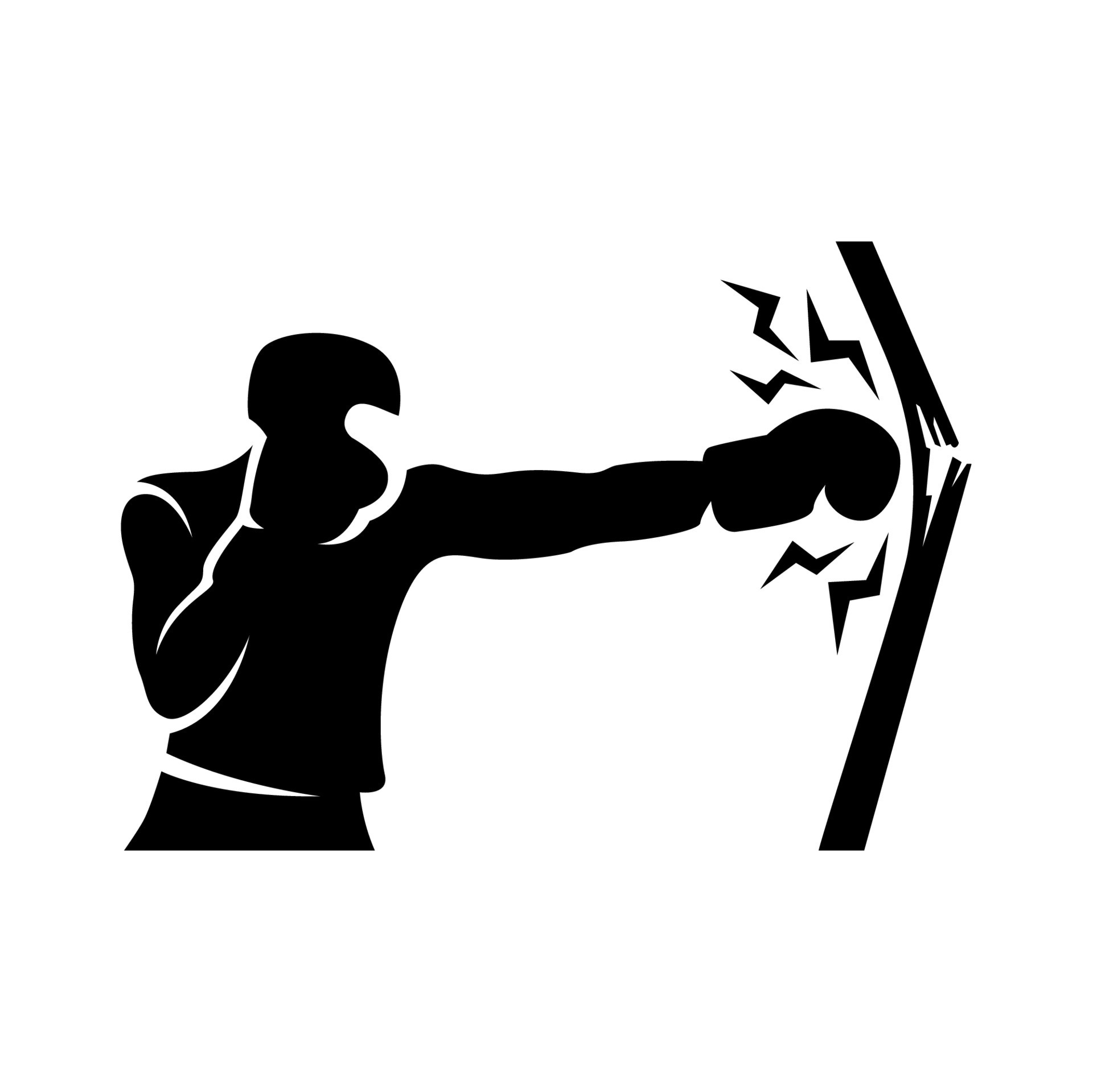The image presents a detailed black silhouette of a boxer set against a stark white background. The boxer is adorned in a black helmet, which leaves the eye area revealed, and is clad in a black shirt and matching black pants. His hands are encased in black boxing gloves. A dynamic action scene is captured, with the boxer delivering a powerful left jab to a black, wooden surface, which is visibly cracked at the impact point. Surrounding the fist is a design depicting lightning-like lines, emphasizing the sheer force and energy of the punch. The silhouette offers a striking contrast with the white backdrop, highlighting the boxer's formidable stance and the intense moment of impact.